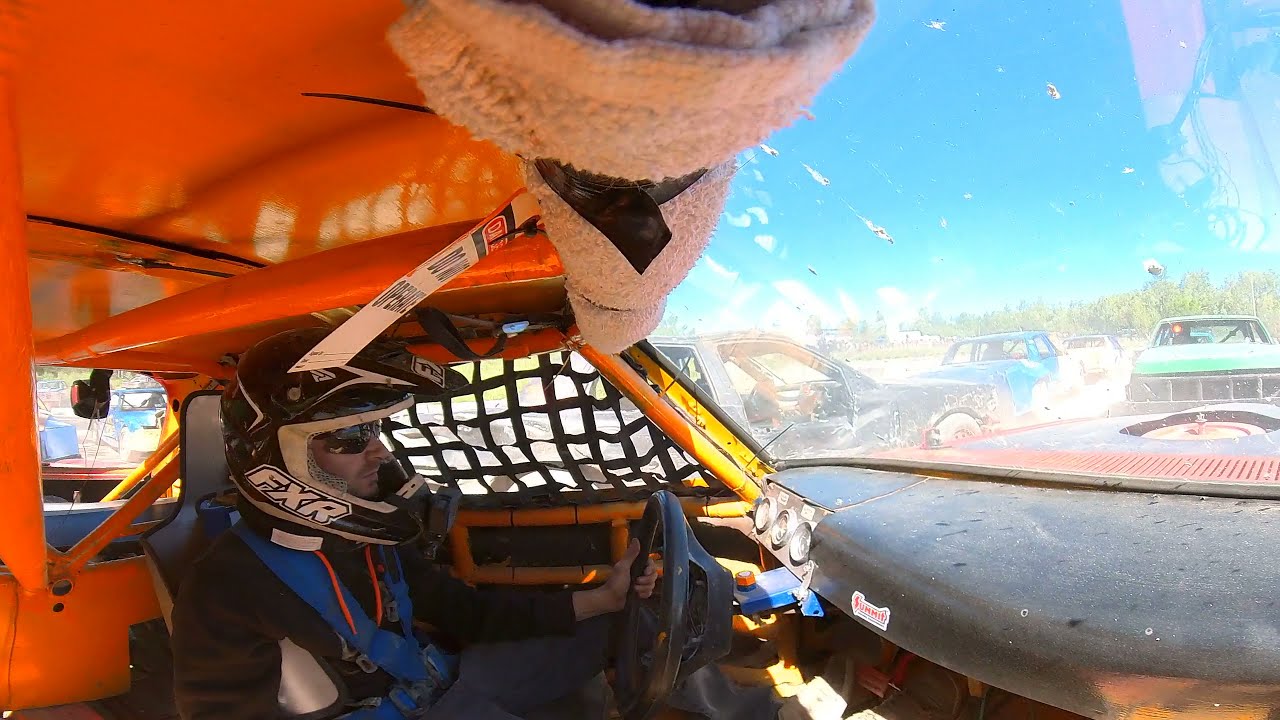Inside a rugged, bright neon orange rally car, a man steers the vehicle, which faces right in the image. The interior is minimally designed with bare metal panels and roll bars that have been spray-coated orange and padded with cloth towels for extra protection. The driver, dressed in black clothing accented with neon blue straps, dons a futuristic racing helmet with black sunglasses. He grips a small steering wheel that protrudes from the dash. On the driver's side window, there’s black plastic netting, and the windshield above, slightly dirty from a muddy course, is topped with cloth padding for additional safety.

Outside, the scene unfolds with several cars parked along a line, depicting a mishmash of amateur scrap vehicles, some missing doors and covered in mud, indicating they've been through rough, industrial races. A green car sits closest to the orange vehicle, followed by a blue one. The sky overhead is an unusual neon teal color, contrasted by green plants visible further back behind the parked vehicles. The atmosphere suggests a gritty, real-world rally event without any visible text or signage.